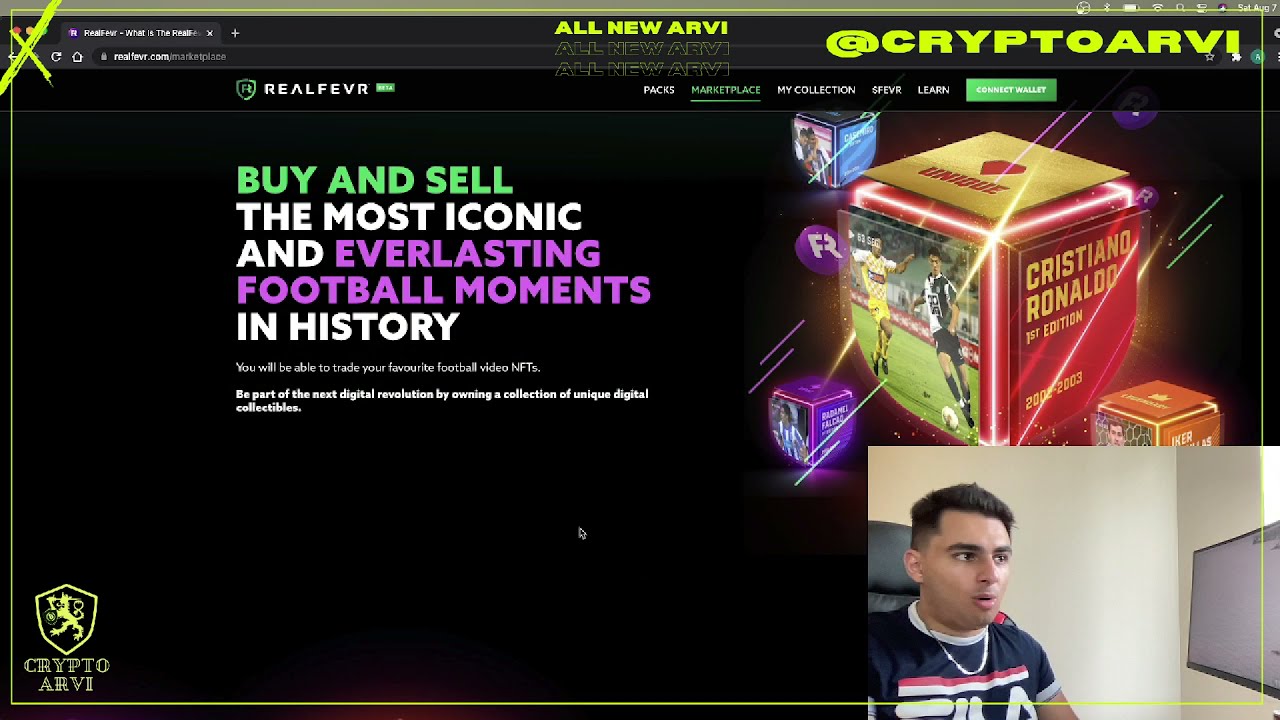The horizontal rectangular image is a detailed computer screenshot against a black background. At the center-left, five lines of text left-aligned read: "Buy and sell the most iconic and everlasting football moments in history." Key phrases "Buy and sell" are highlighted in green, "everlasting football moments" in purple, while "the most iconic" and "in history" are in white. Below this text is smaller, less legible text. In the lower left corner, there's a gold badge logo with the text "Crypto RV" underneath it. In the lower right corner, a man wearing a blue, red, and white striped Fila T-shirt, accessorized with a necklace, is visible, looking at a computer monitor. In the upper right corner, there's additional text in yellow that says "@Crypto RV." Adjacent to this is an image resembling a cube, featuring the words "Cristiano Ronaldo, first edition" in gold with a red background on one face, and images of soccer players on other faces. The context appears to be a webpage from the platform Real Fever, offering a service to buy and sell iconic football moments. The overall theme suggests a digital marketplace for football memorabilia, intersecting technology and sports history.